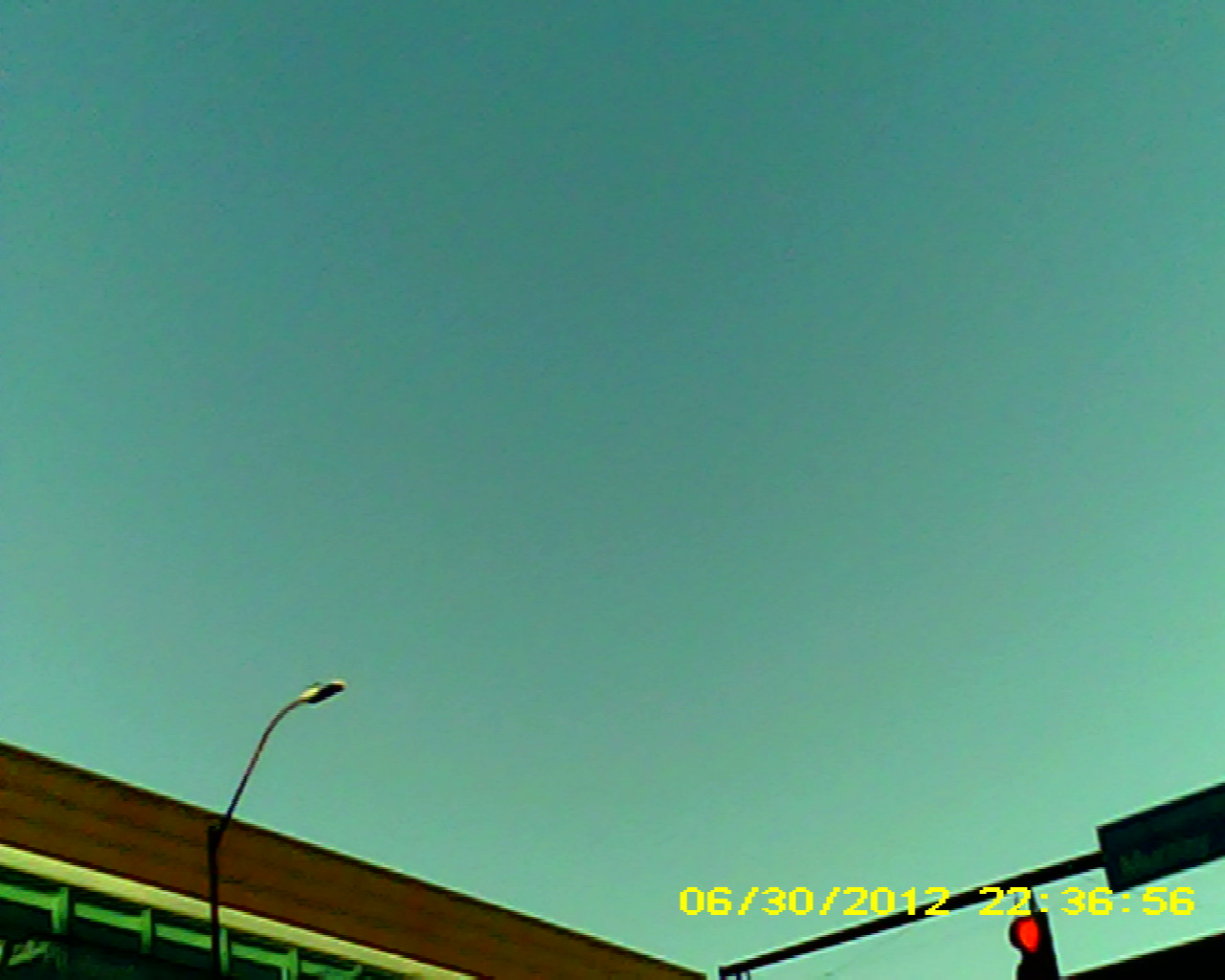This dash cam or street camera image, dated June 30th, 2012, captures a scene at 22:36:56 (military time) which is late evening. However, the sky appears unusually bright, resembling daylight. The bottom left corner of the frame features part of a building, and nearby, a street lamp stands tall. At the intersection seen in the image, a red traffic light is visibly illuminated, adding context to the urban environment.